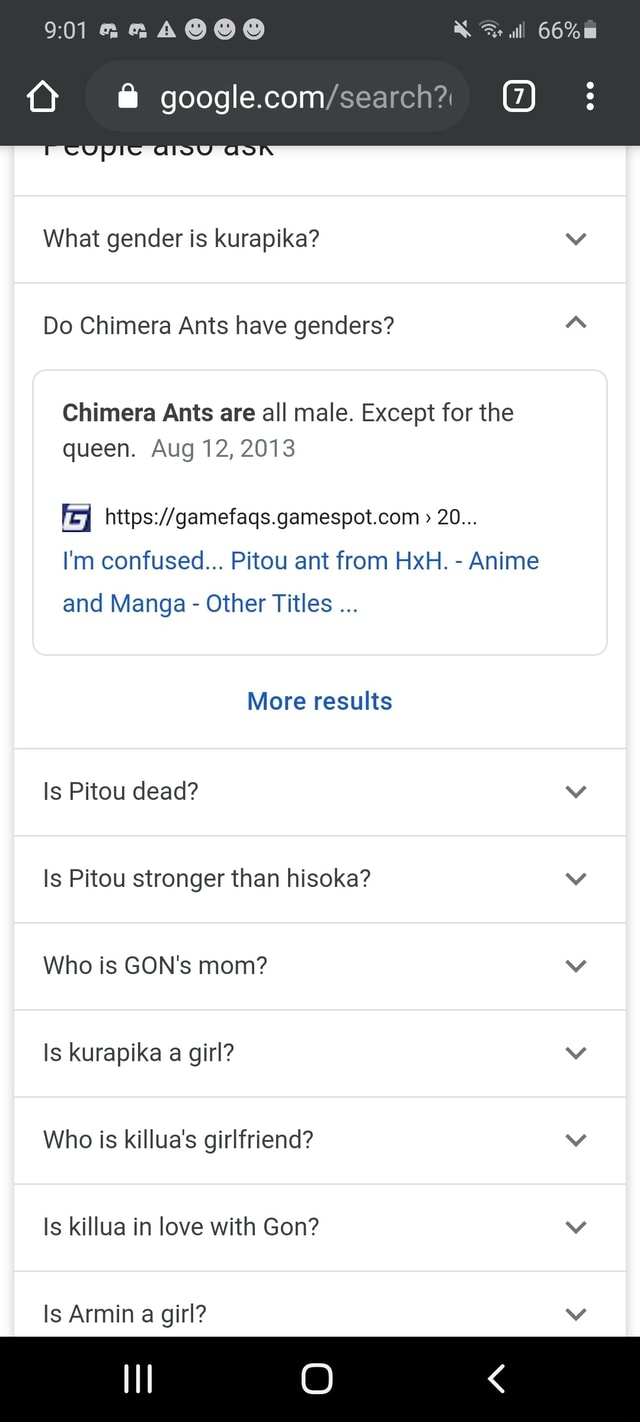The image depicts a smartphone screen displaying a web browser open to a search engine query. The phone's status bar at the top shows a battery life of 66% and the current time as 9:01 AM. Alongside the time and battery indicators, the status bar also includes a series of emoji icons—primarily smiley faces and possibly a crying face—creating a black bar across the top.

The browser is open to "google.com" with a search box at the center of the screen containing a query about Chimera ants and Kurapika. Beneath the search bar are options for a Home icon, a lock icon, a box containing the number seven, and three vertical dots indicating a menu.

Displayed prominently is a section titled "People also ask," featuring a variety of questions related to anime topics. Some of the visible questions include:
- "What gender is Kurapika?"
- "Do Chimera ants have genders?"

A pop-up appears providing information that states, "Chimera ants are all male except for the queen," dated August 12, 2013. It also mentions a character named Pito from the "H×H" anime and manga series.

Further down, a button labeled "More results" in blue invites users to see additional inquiries such as:
- "Is Pitou dead?"
- "Is Pitou stronger than Hisoka?"
- "Who is Gon's mom?"
- "Is Kurapika a girl?"
- "Who is Killua's girlfriend?"
- "Is Killua in love with Gon?"
- "Is Armin a girl?"

At the bottom of the screen, a black navigation bar displays three vertical lines, a Home icon, and an arrow pointing to the left.